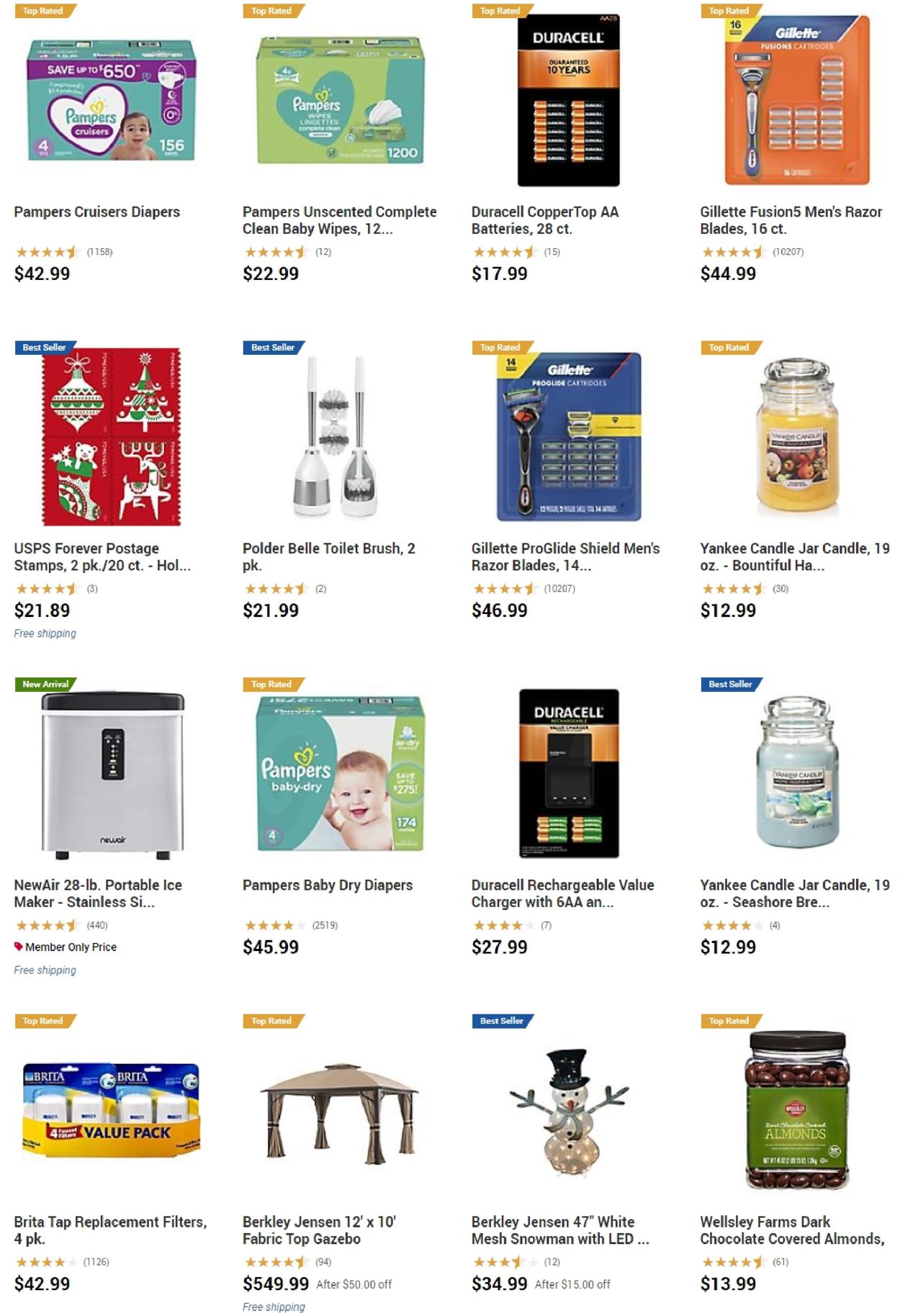The image showcases a Costco webpage featuring several highly-rated products for sale. Dominated by top-rated orange banners, the page highlights various items including:

- **Pampers Cruisers Diapers**: Priced at $42.99, these diapers come in a brightly colored package featuring teal, purple, and white hues.
- **Pampers Cruisers Unscented Complete Baby Wipes**: A green and light green package priced at $22.99, also marked as top-rated.
- **Duracell AA Batteries**: A 28-count package priced at $17.99, tagged as top-rated.
- **Gillette Fusion Men's Razor Blades**: Displayed in bright orange and blue packaging, these blades are priced at $44.99 and are top-rated.
- **Forever Stamps (Christmas Design)**: A 20-count set priced at $21.89, marked as a best seller with free shipping.
- **Toilet Brush**: Priced at $21.99 and marked as a best seller.
- **Additional Gillette Shavers**: Priced at $46.99.
- **Gazebo Tent**: A top-rated brown gazebo tent priced at $549.99.

Each item is visually distinct, with vivid packaging and prominent banners indicating their high ratings and best-seller status.